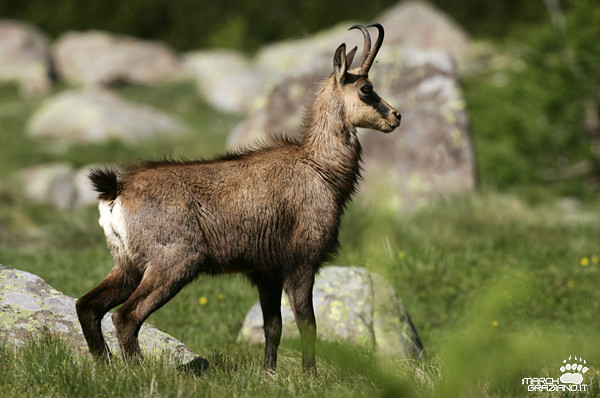The photograph showcases a mountain goat standing in a grassy outdoor landscape. The goat, viewed from its right flank, occupies the left side of the image while gazing to the right. Its medium-length brown fur varies in shades, featuring a small, bushy black tail and a white rump. The animal boasts two prominently curved horns that resemble fish hooks, arching back towards its head, and its perked ears add alertness to its demeanor. The scene is replete with natural elements: the immediate foreground includes thick green grass, and behind the goat are a few large, light gray boulders with more scattered rocks visible in the background. The upper right corner of the image displays some indistinct shrubbery, adding depth to the wilderness setting. Adding a touch of professionalism, the bottom right corner of the photo contains a white watermark, resembling an animal footprint, alongside the text "March Grozenoyte," a blurry logo that seems imprinted on top of the image.